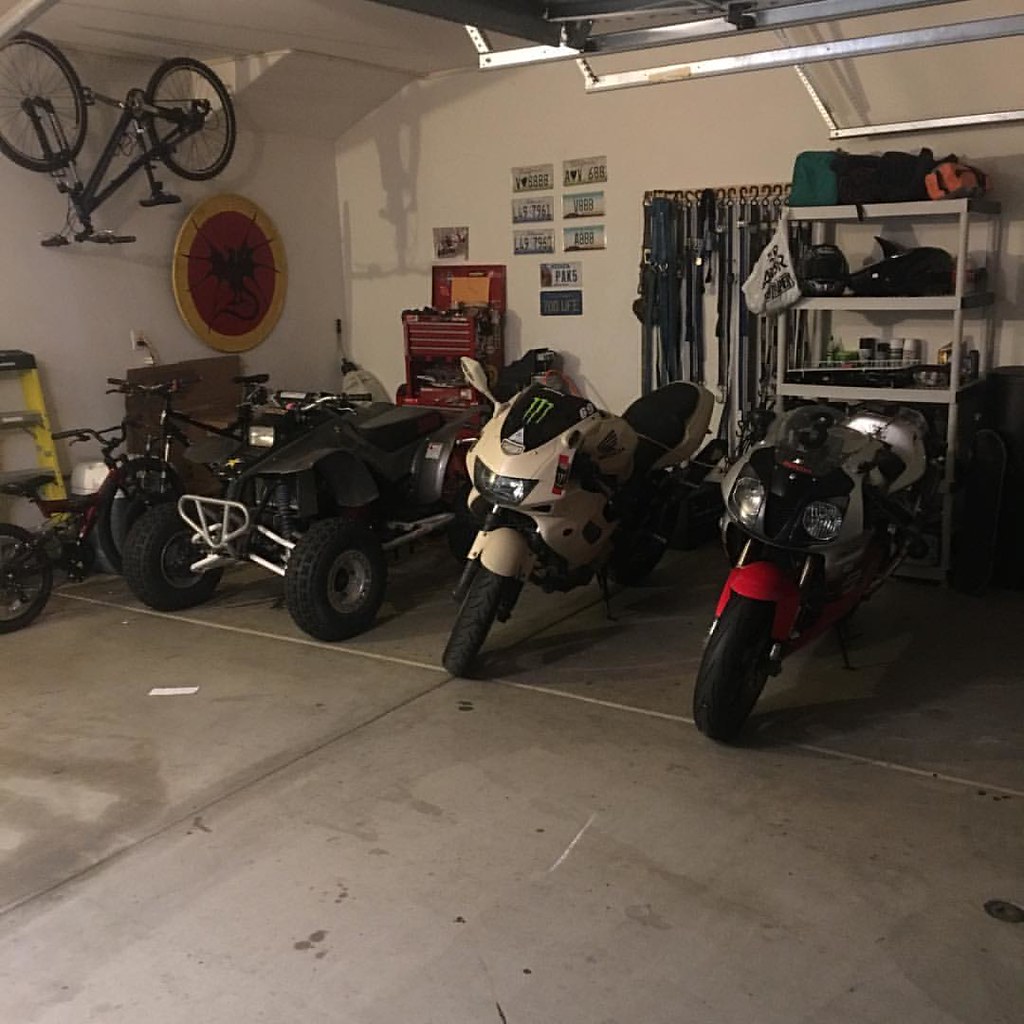This dimly lit photograph captures the cluttered interior of a garage with a concrete floor and white walls. Suspended from the ceiling on the left side is a black bicycle. Various equipment and objects fill the space, including two bicycles parked on the floor. The back wall is adorned with multiple license plates, and a red toolbox sits prominently. A shelving unit holds items like paint cans and helmets, while a rack on the wall displays an array of belts and bungee cords. Also notable in the garage are an ATV and two motorcycles—one white and the other black and red. In the background, there's an emblem featuring a dragon, adding to the eclectic decor. The garage door is visible, raised upwards, hinting at the space's utilitarian nature.